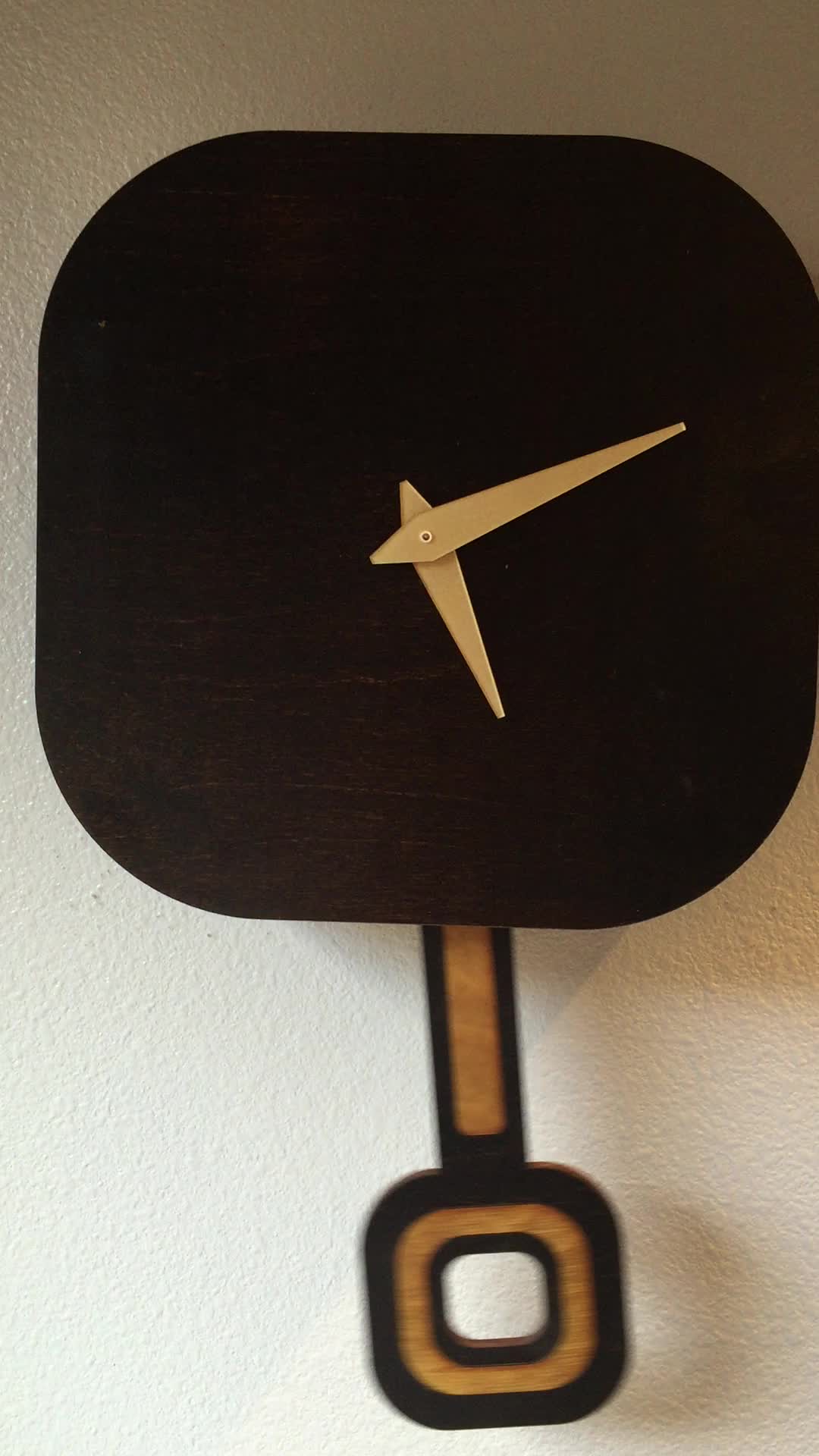In this vertically oriented photograph, a clock is mounted on a textured white wall. The clock features a minimalist design with a completely black face, devoid of any numbers or markings. Both the hour and minute hands are gold, indicating the time as approximately 5:13. Below the clock, a black and brown pendulum hangs, adding a touch of classic elegance to the modern design. The lighting in the image originates from the bottom left corner, casting shadows toward the upper right portion of the wall, creating a dramatic contrast that highlights the clock's simplistic yet striking appearance.